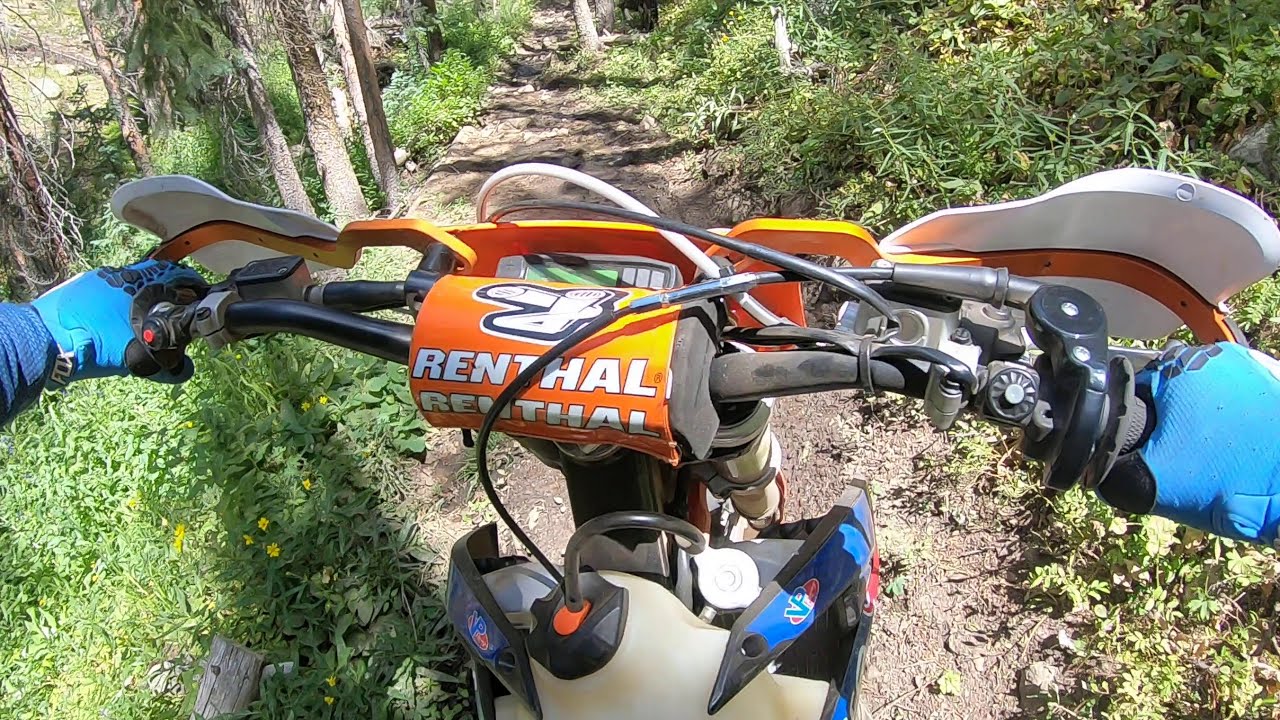The image captures a dramatic off-road mountain biking scene from the rider's perspective, likely taken with a GoPro mounted on their helmet. The bike is navigating a very rocky and muddy trail, surrounded by thick green vegetation and yellow flowers. Sparse, dormant trees with brown trunks and branches add to the rugged terrain. The rider grips black handlebars adorned with light blue gloves that feature black accents around the thumbs and fingers. Centered on the handlebars is an orange cushion bearing the brand name "Renthal" in white letters. An orange bar and white shields are also part of the bike's front assembly, providing additional protection. The trail below is muddy and treacherous, challenging the rider as they make their way up the mountainous path.